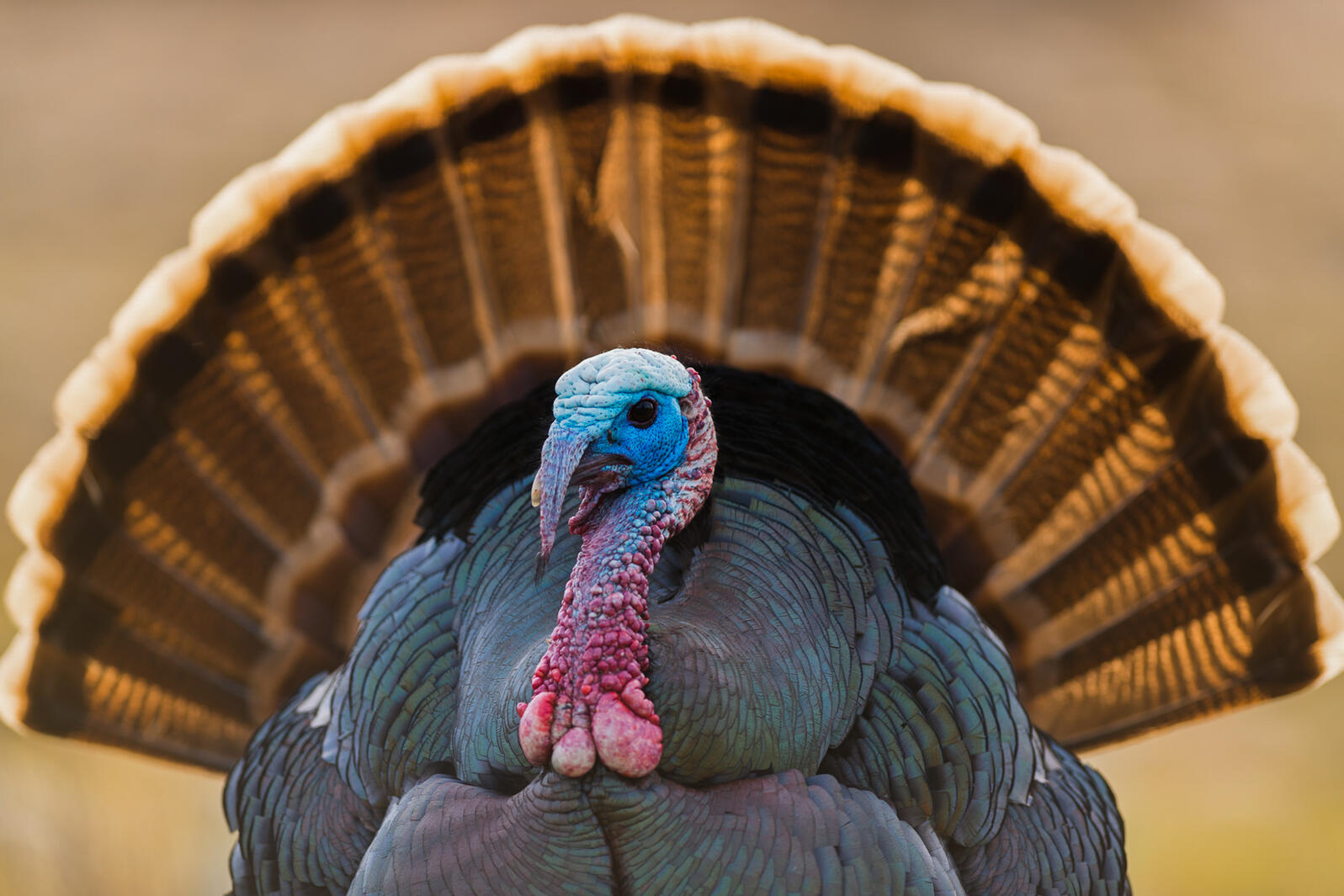This is a detailed close-up photograph of a turkey, centered in the middle of the image. The background features a light brown, marble-like texture that contrasts with the vibrant colors of the turkey. The turkey's face is mostly blue with a red wattle, known for the fleshy part hanging down its neck, which is pinkish in color with three white knobs at the end. Its head is topped with a white crown, and you can see one visible black eye under part of the red wattle that obscures the other eye. The body of the turkey is grayish-blue with a multitude of lines giving it a billowy appearance. The intricate tail feathers spread out in a semicircular fan behind the body, taking up a significant portion of the background and fading into a blur. These feathers showcase a striking pattern with brown, orange, black, and white strips that include black edges and white tips at the end. Additionally, there are black line drawings adjacent to the turkey's head that resemble hair. The overall composition and color contrasts make the turkey the clear focal point of this fascinating and detailed image.